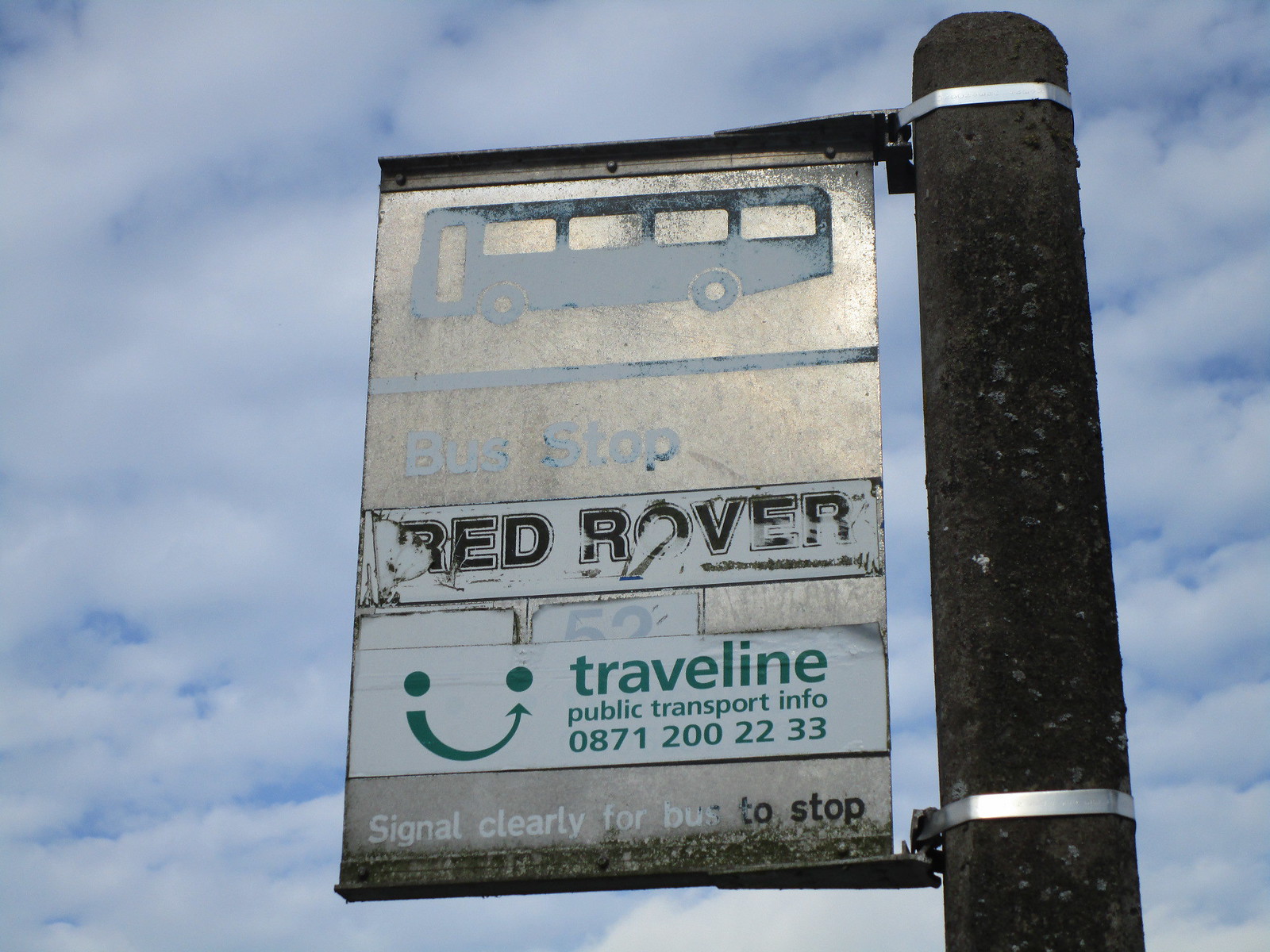A dilapidated bus stop sign stands affixed to a rusty, dark grey pole on the right, secured by two metal rings. The sign is weathered and faded, with its paint peeling away to reveal a silvery layer beneath. At the top of the sign, a blue icon of a bus with four windows faces left, partially reflecting light from the sun above. Below the bus icon, the words "bus stop" are barely legible in faded blue text, followed by "Red Rover" in black font and a sticker indicating Route 52. The sticker reads "travel line, public transport info 0871 200 22 33" and instructs passengers to "signal clearly for bus to stop." In the background, a sky filled with mostly faded white clouds completes the scene, contrasting with the grody appearance of the sign and pole.